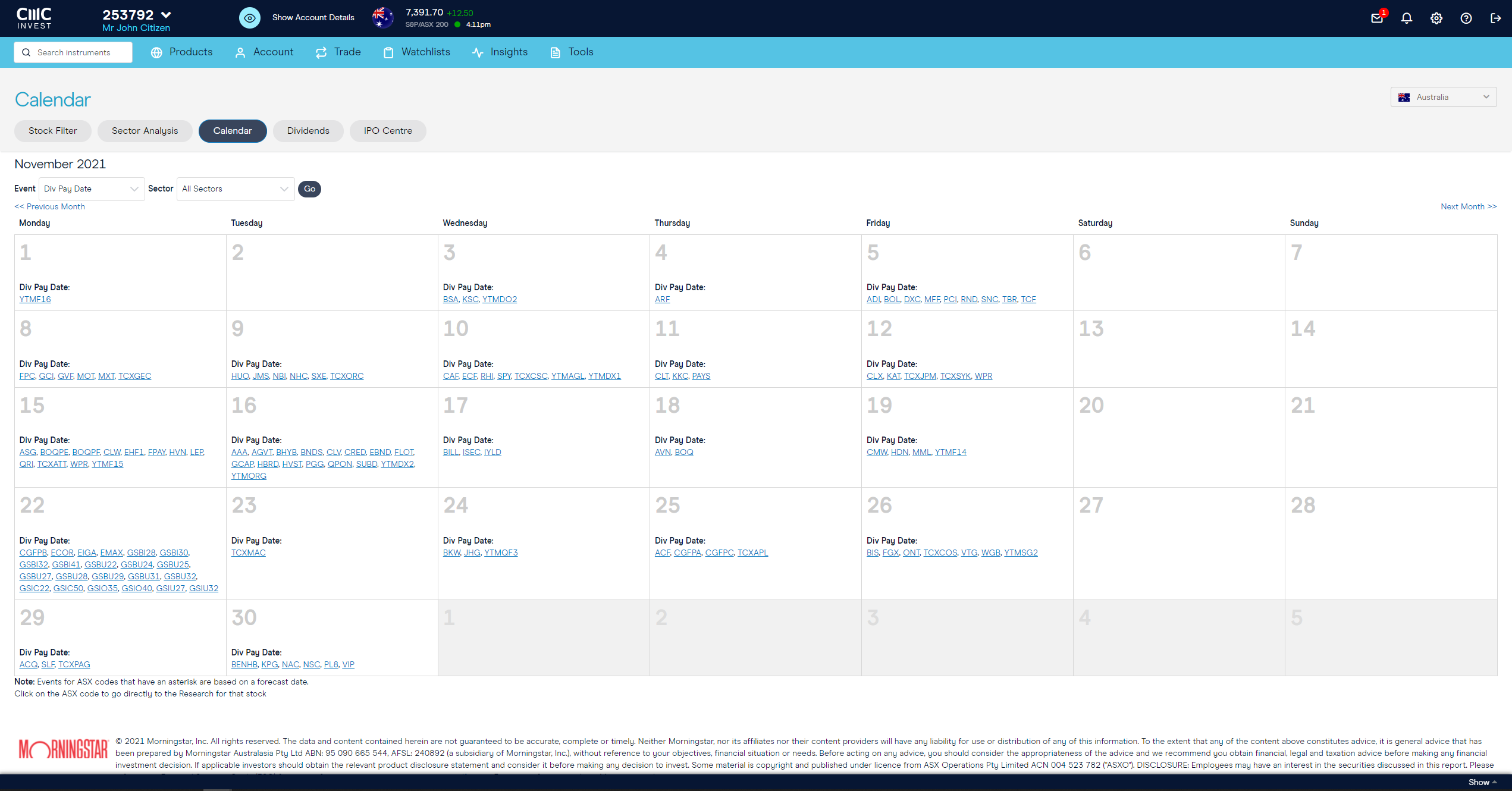A detailed screenshot from a website titled "See CC Invest," prominently displaying the name "Mr. John Citizen" and the user account number "253792." Beneath an eye icon labeled "Show Account Details," a circular graphic featuring the British flag announces a balance of "7391.70" in green, indicating an increase of "12.5." Lower down, a calendar featuring November 2021 is filled with clickable blue links and underlined dates. Highlighted on Monday, the 1st, is a file labeled "Y TMF 16." The bottom section of the screenshot features the Morningstar logo with the text "© 2021 Morningstar Incorporated. All rights reserved," and finishes with a paragraph describing the company, all enclosed within a black rectangular footer.